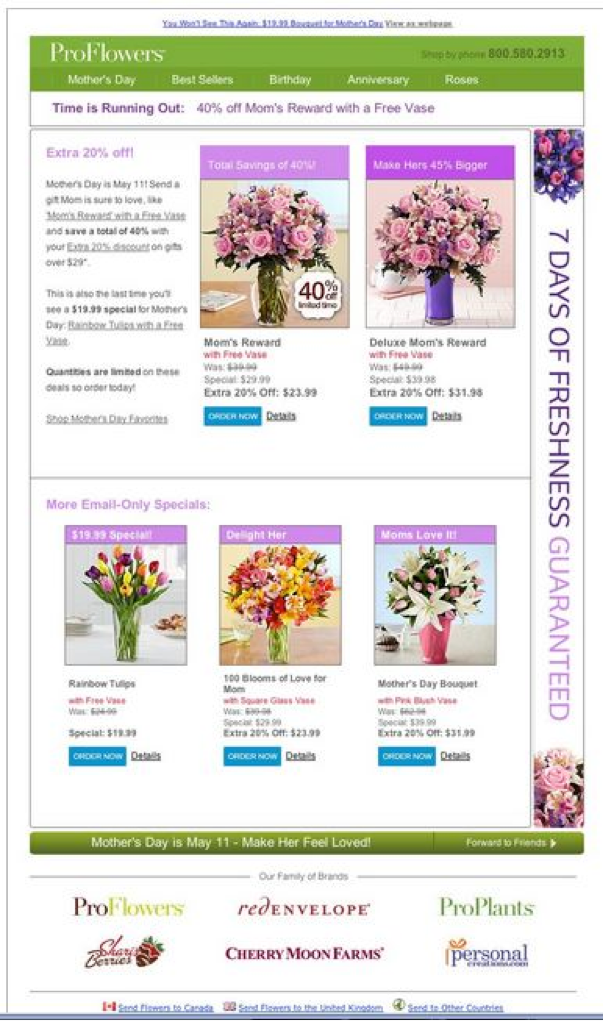The website in question is ProFlowers, which features a predominantly green-themed header resembling the shades of a leaf transitioning to an olive green. The logo reads "ProFlowers," with the 'P' from "Pro" and the 'F' from "Flowers" capitalized. Adjacent to the logo, there's a contact number for ordering: 800-580-2913. Directly below, the navigation bar includes categories such as Mother's Day, Best Sellers, Birthday, Anniversary, and Roses.

A prominent message in purple text states, "Time is running out! 40% off Mom's Rewards with a free vase." This announcement is arranged in three vertically stacked rectangles. Just below these, another rectangle advertises an additional 20% off, emphasizing the urgency by noting that Mother's Day falls on May 11th. It encourages customers to send a gift mom will adore, offering items like the "Mom's Reward with a free vase," now at a total discount of 40% on orders over $29. There's also a specific mention that this will be the last time the $19.99 special for Mother's Day Rainbow Tulips with a free vase will be available, highlighting the limited quantities and urging immediate purchase. A link labeled "Shop Mother's Day favorites" enables further browsing.

Beneath this information, two images of flowers are displayed. The first image shows pink flowers in a clear white vase on a wooden table beside a magazine, with a window and tan wall in the background. The caption indicates a total saving of 40%, with the "Mom's Reward with Free Vase" originally priced at $39.99, now on special for $29.99, and further reduced to $23.99 with an extra 20% off. There are "Order Now" and "Details" buttons beneath this offer.

The second image features flowers in a purple vase with the tagline "Make hers 45% bigger." This is the "Deluxe Mom Reward with Free Vase," initially priced at $49.99 but reduced to $39.98, and further discounted to $31.98 with the extra 20% off. It also includes "Order Now" and "Details" buttons.

Flanking these images, side bars with text in purple assert a "Seven Days of Freshness GUARANTEED." Additionally, an email-only special features Rainbow Tulips with a free vase, originally $24.99, now $19.99, accompanied again by "Order Now" and "Details" options.

Further down, another featured product is the "Delight Her: 100 Blooms of Love for Mom" in a square glass vase, discounted from $39.99 to $29.99, with an additional 20% off pricing it at $23.99. This section also includes options for ordering and viewing more details.

Lastly, the "Mom's Love it Mother's Day Bouquet with Pink Blush Vase," initially priced at $42.99, is available for $39.99, further reduced to $31.99 with the extra discount. It also provides "Order Now" and "Details" buttons.

At the bottom, an olive green bar reiterates that Mother's Day is May 11th and urges customers to make their moms feel special. There's a clickable "Forward to Friends" button followed by links to other brands under the ProFlowers family, such as Red Envelope, ProPlants, Cherries Berries, Shari's Berries, and Personal Creations, among others. The page also includes options to send flowers to Canada, the United Kingdom, and other countries.